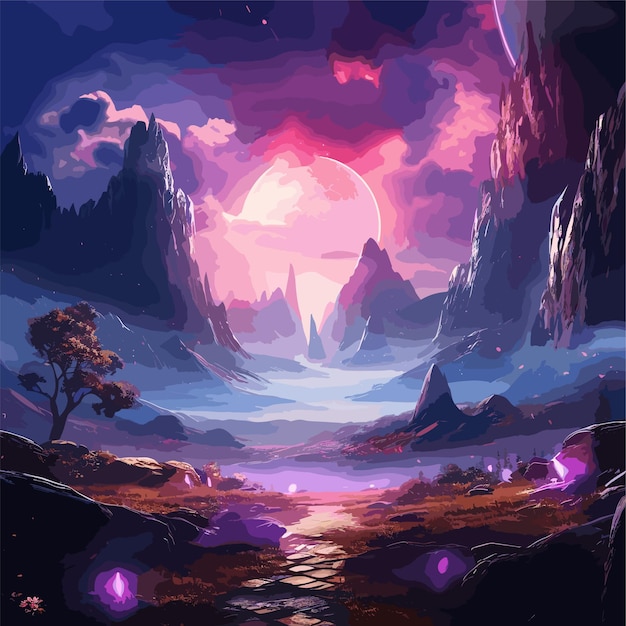The image captures a vibrant, digitally illustrated fantasy landscape with a painterly aesthetic. Dominating the background are towering, sharp mountain peaks under a sky infused with hues of purple, pink, and tan, reflecting light—likely from a partially obscured celestial body, possibly a moon. The transitioning sky gives way to the ground, which is primarily brown and semi-arid, dotted with a hint of water reflecting the moonlight. Small, glowing purplish-violet creatures with halos add a sense of mystery and sci-fi flair to the scene. The middle ground features a river or lake nestled between the rocky formations, leading to a path that crosses the landscape. A solitary tree stands on the left, surrounded by small, enchanting, glowing objects that resemble fireflies. The overall scene suggests an uncharted, possibly extraterrestrial world, blending natural elements with a whimsical, otherworldly ambiance.